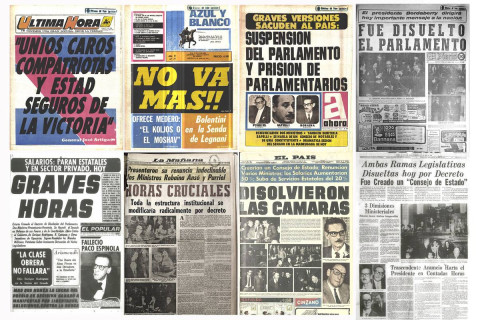The image depicts a collection of eight old newspaper pages or possibly magazine pages, likely in Spanish, arranged in two rows—four on the top and four on the bottom. The majority of the pages are black and white, featuring large headlines and black and white photographs. However, the first three pages in the top row are in color: the first one includes blue, pink, and white; the second one features blue, orange, and yellow; and the third has some yellow on it. Each page seems to focus on one or two main articles, many of which are front pages judging by the prominent headlines. Notable headlines include "No Va Más," "Fue Disilento el Paramento," "Oras Cruciales," and "Greves Oras." These newspapers likely cover similar topics, as seen in the repeated use of the word "oras." The headlines also include phrases like "Última Hora no caros con perritos y esta seguros de la victoria" and "Suspension del Parlamento," suggesting the coverage of significant events. The layout and detailed presentation of the pages indicate a historical and possibly significant array of journalistic efforts.